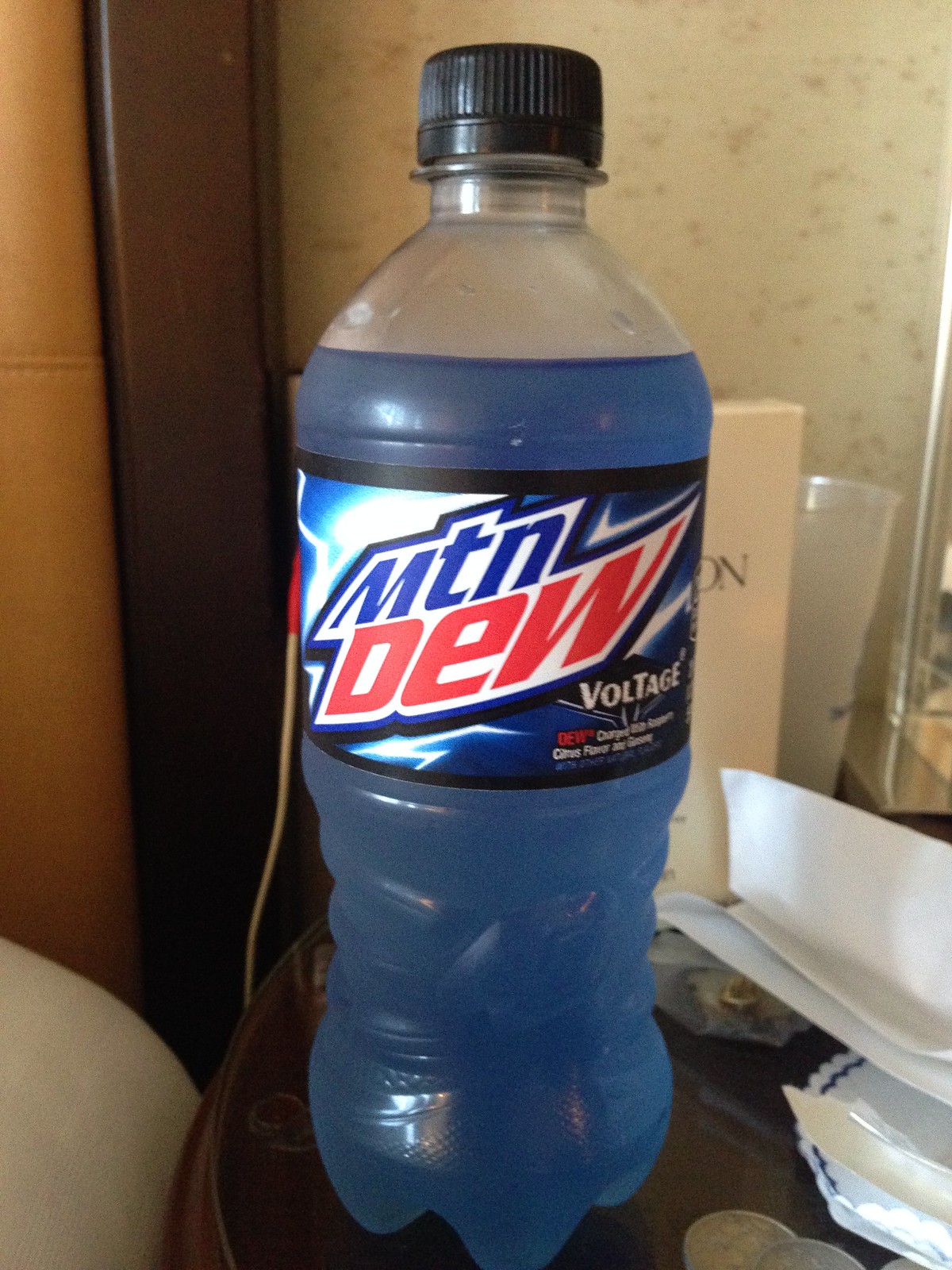In this photograph, the most prominent object is a bottle of Mountain Dew Voltage. The bottle contains a vibrant blue liquid and is made of clear plastic, topped with a black cap. The label on the bottle features a striking blue lightning bolt design, with the word "MTN" displayed in bold blue font, "Dew" in eye-catching red font, and "Voltage" in crisp white font. The label is accentuated with black rims at both the top and bottom edges. The bottle rests on a brown table, surrounded by various other items. To the left, there is some white paper and scattered coins. Behind these items, an off-white box is visible, along with a cup situated next to it. A partial view of a wooden frame is also seen, alongside some white material that could be part of a bed frame. In the background, the wall is a tan color with patches of gray discoloration, adding a rustic touch to the scene.